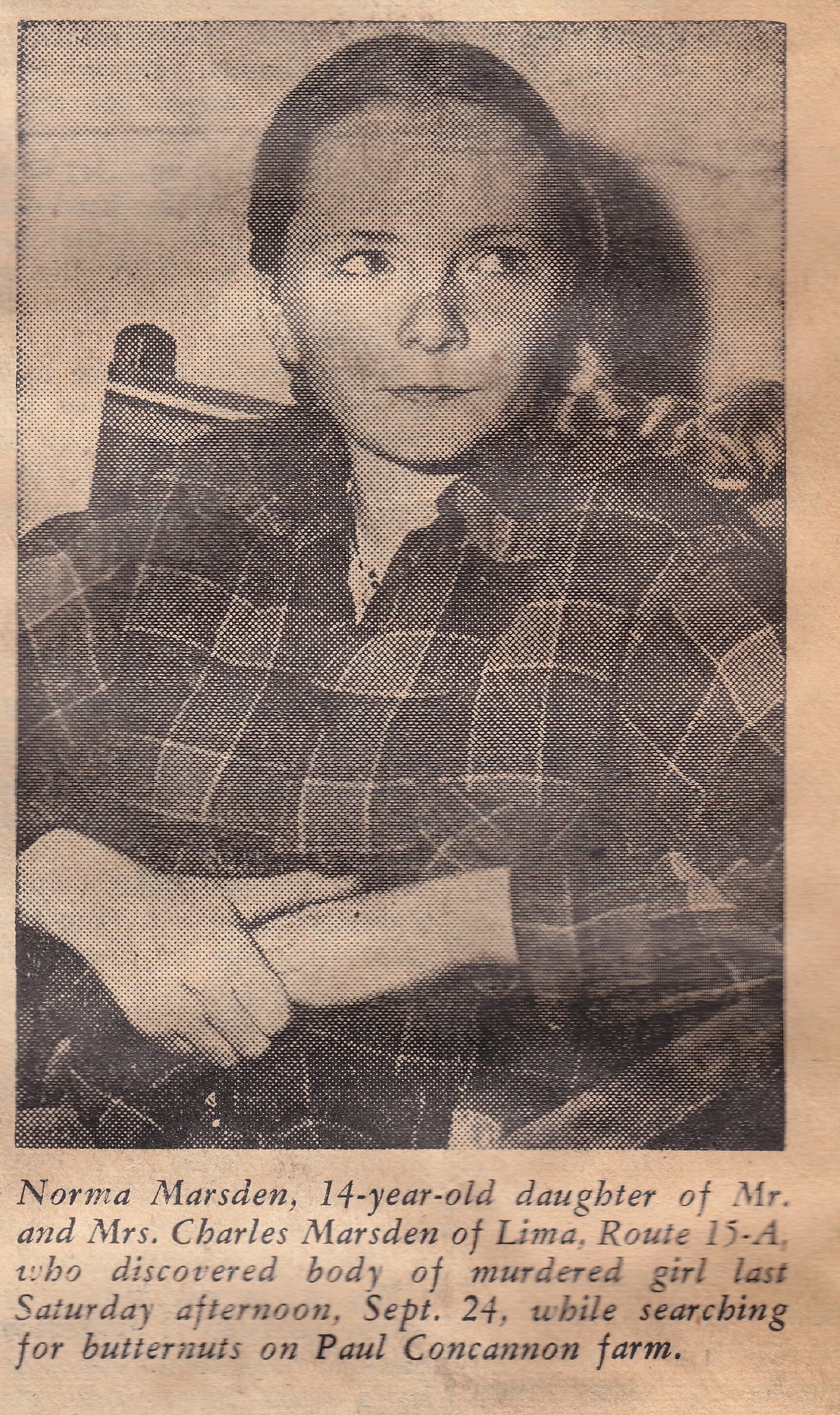This black and white image, likely a snippet from an old magazine or newspaper, prominently features a photograph of a young woman named Norma Marsden. Norma, identified in the caption as the 14-year-old daughter of Mr. and Mrs. Charles Marsden of Lima Route 15A, is described as wearing a plaid shirt and a necklace, with her long blonde hair styled in a braid. She is seated in a chair and gazing off to the right side of the image. The background exhibits shades of tan, black, white, and various grays, giving the sense that the clipping is aged and somewhat worn. Text at the bottom details Norma's discovery of a murdered girl on Saturday, September 24th, while she was searching for butternuts on Paul Kahn Cannon Farm. The overall appearance of the clipping suggests it has faded over time, leaning more toward brownish tones.